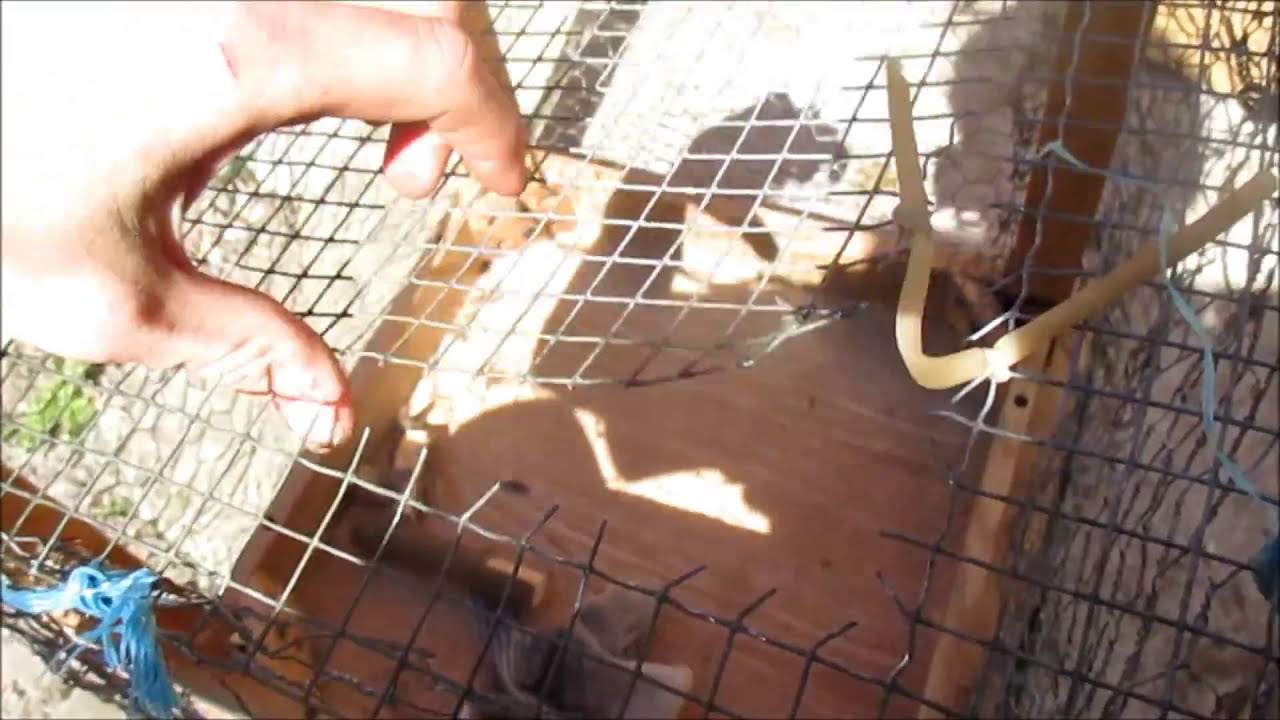The image depicts a detailed scene of a damaged cage, predominantly composed of metal wires resembling chicken wire, which have been crudely cut and peeled back, exposing sharp edges. Emerging from the top left corner, a Caucasian hand reflects bright white light, highlighting a pronounced red scar on the knuckle. The hand's middle finger and thumb grip the jagged metal edges, attempting to widen the opening further, with the fingers partially piercing through the mesh. Below the hand, in the bottom left corner, a piece of blue string is visible, while on the right side, an orange-yellow rubber piece and a light blue string appear to be loosely securing the cage. The cage itself is supported by a wooden frame and base, hinting at a constructed animal enclosure, possibly for birds. The wooden floor beneath, along with wooden railings, fortifies its structure. The overall scene suggests intrusion and damage, further hinted by the wire's L-shaped cut, creating an atmosphere of abandonment or escape from the cage. In the midst of the metal mesh, there’s a fleeting glimpse of what might be the body of a bird, although its head is obscured, adding to the uncertainty within the confines of the cage.